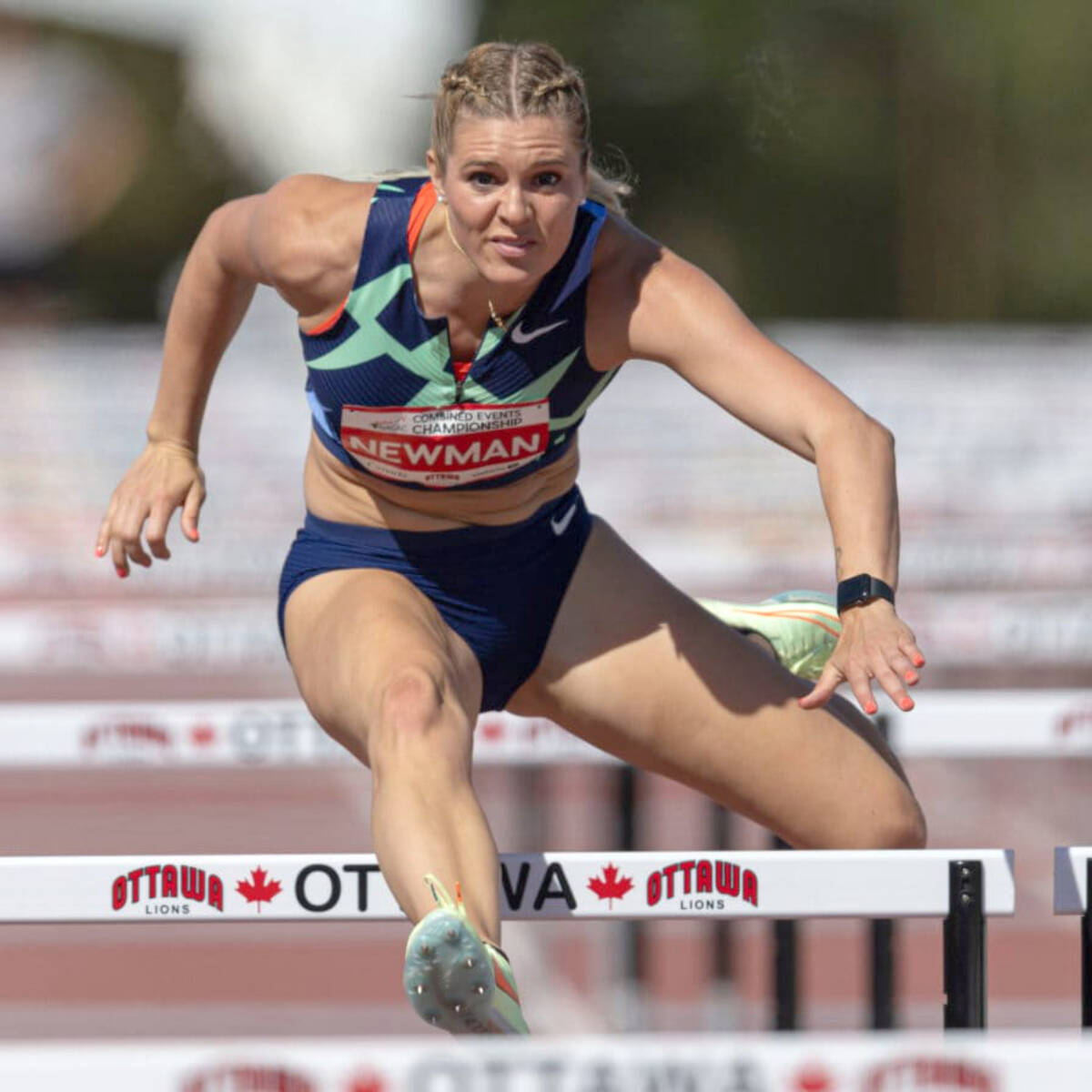The photograph features a determined young woman in her 20s with light-colored skin and dirty blonde hair styled in two French braids. She is captured mid-air while jumping over a white hurdle adorned with "Ottawa" and "Lions" in red and black text, flanked by red maple leaves, indicating the event is taking place in Canada. The background is slightly blurred with hints of green and indistinct shapes of hurdles. The athlete exudes strength and focus, her blue tank top with green and orange accents and matching blue shorts prominently displaying the name "Newman" on a red banner on her chest. Both her top and shorts feature the Nike logo, and she is equipped with a black Apple watch on her left wrist. Her poised, muscular frame is accentuated by the intensity of her leap, her right leg almost clearing the hurdle while her left leg trails behind. Her arms are outstretched for balance, and her meticulously manicured coral-colored nails add a touch of elegance to her powerful, athletic presence.